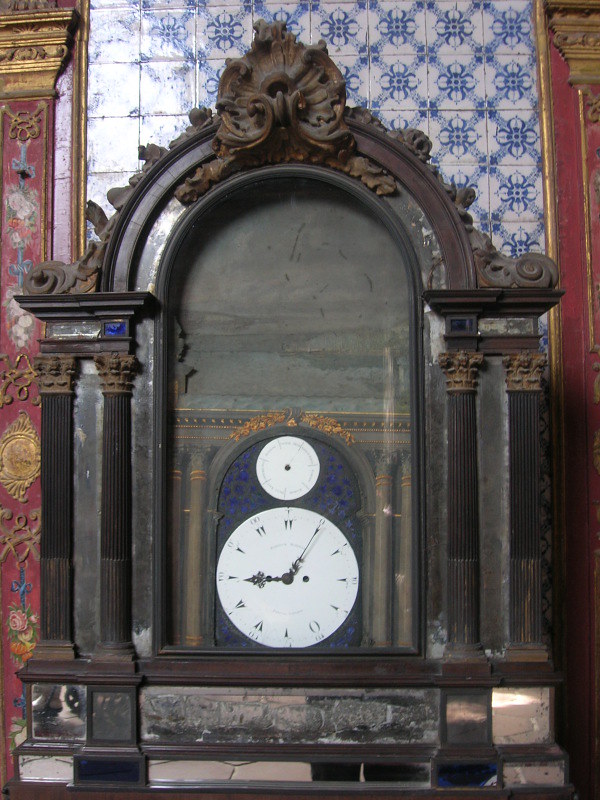The image showcases an antique clock, prominently placed at the center. The clock is encased in a brown wood frame, exuding a rich, vintage aesthetic. The top of the frame is notably ornate, adorned with intricate carvings and an elegant arch design. Surrounding the clock is a mirrored trim, which shows visible signs of age and wear, particularly on both sides beneath the arch.

The clock's structure includes a flat-topped column flanked by two fluted columns, all in matching brown wood. The central arch inside the frame features a decorative blank upper section and a supplementary arched area below, housing the clock face.

The clock face is striking in design, with a clean white background, black hour and minute hands, and Roman numerals marking the hours. Above the main clock face is a smaller, less readable circular component. Adjacent to the clock face, on either side, are additional fluted columns, enhancing the ornate appearance of the clock.

The detailed craftsmanship and the inclusion of fluted columns and mirrored trim suggest a blend of traditional design elements with signs of aging, indicating this could potentially be generated through advanced computer graphics, mimicking an authentic antique look.